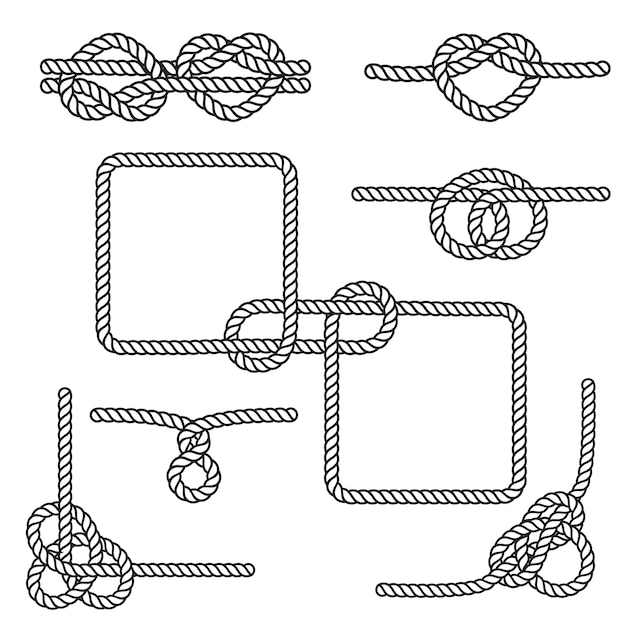This black-and-white, hand-drawn diagram features seven aesthetically arranged, somewhat complicated knots formed by ropes. Each knot type is neatly positioned within the square frame of the image, creating pleasing corners with the largest and most prominent knot centered. The illustration is devoid of any text or instructional information, focusing purely on the visual representation of the knots. Some knots appear to have heart shapes, notably at the top, with others resembling pretzels or simple twists. The central knot, unique in appearance, seems possibly impossible given its lack of visible rope ends. While seemingly a digital representation, the detailed diagram maintains an arts-and-crafts instructional style, suggesting it could belong in an educational book on knot tying.